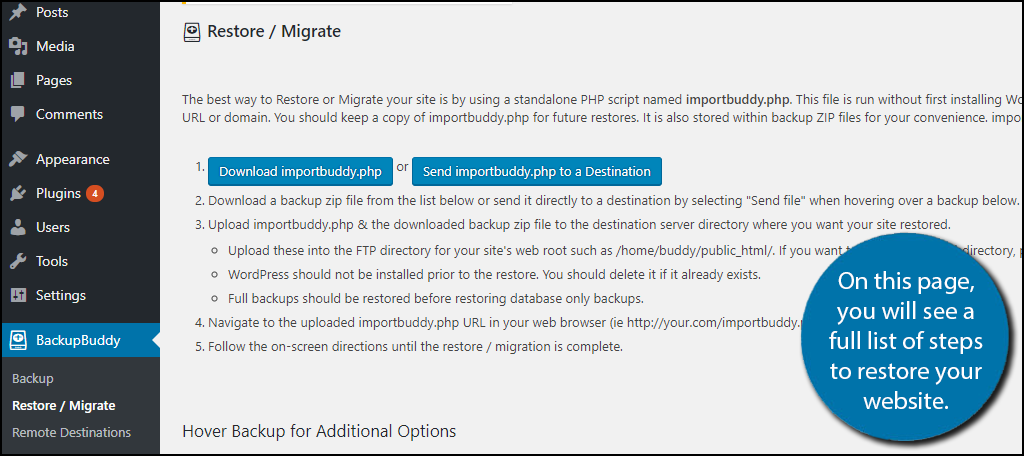This is a screenshot of the Backup Buddy app interface. On the right-side menu, there are various tabs labeled "Post," "Media," "Pages," "Comments," "Appearance," "Plugins," "Users," "Tools," "Settings," "Backup Buddy," and a section called "Restore/Migrate." Below this menu, there is an option called "Remote Destinations," indicating the current section is focused on Backup Buddy.

The main content area above displays a header titled "Restore/Migrate" with a description stating, "The best way to restore and migrate your site by using a standard PHP script named ImportBuddy.php." The text explains that this file can be run without first installing any additional software and emphasizes the importance of keeping a copy of ImportBuddy.php for future use. To the left, there is a circular icon that presumably provides more details. On the right side, the text mentions that this page provides a complete list of steps necessary to restore your site.